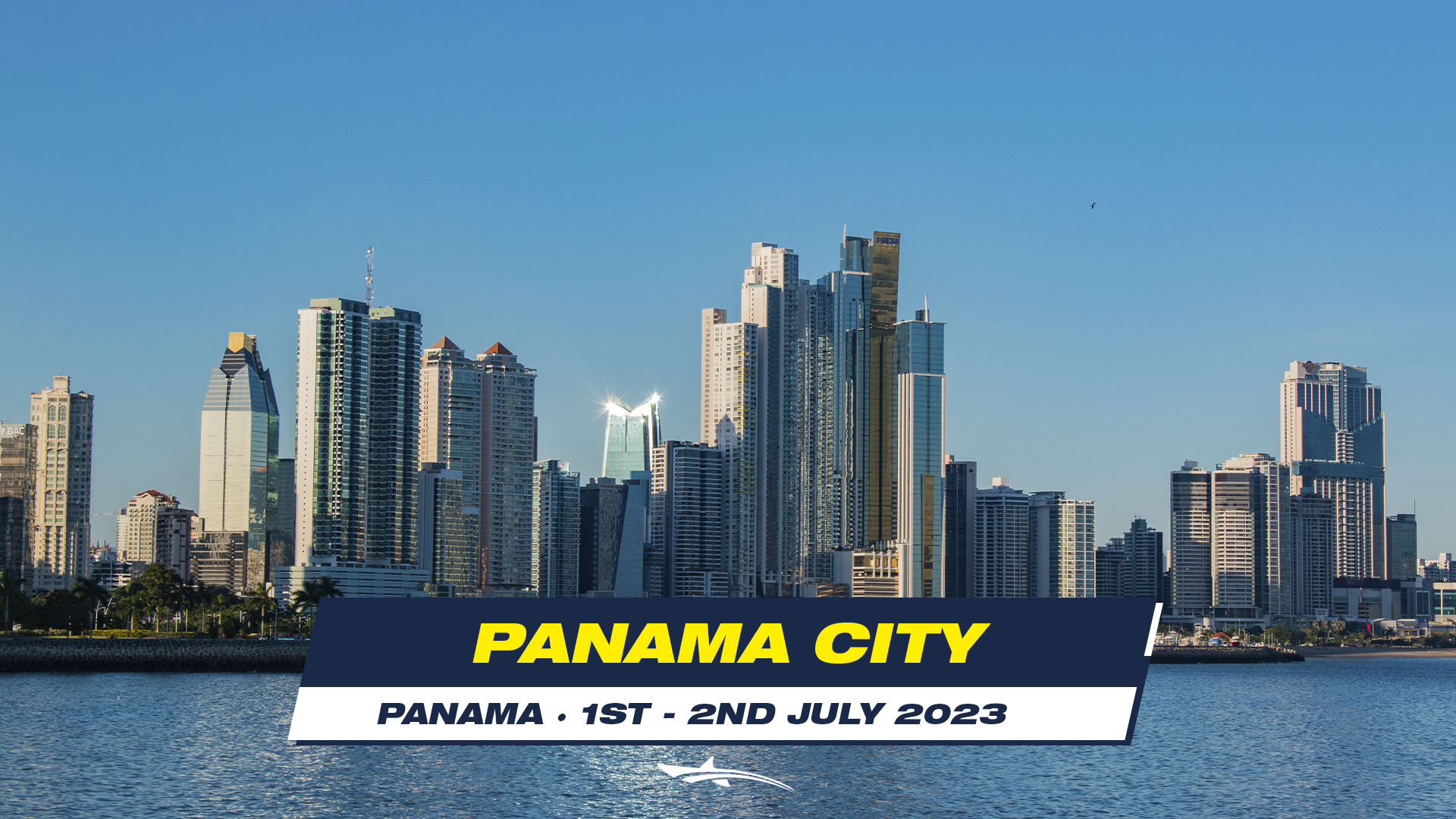The image features a clear blue sky that gradually lightens towards the horizon, serving as a vibrant backdrop for a modern city skyline dominated by towering skyscrapers. These buildings, mostly appearing to be contemporary apartment complexes, rise impressively against the sky. Closer to the camera, lush green trees provide a natural contrast to the urban landscape. In the foreground, a body of water adds a serene element to the scene, with a ship docked at the bay. Prominently displayed in bold yellow capital letters against a dark blue background are the words "PANAMA CITY." Directly beneath this, a white box contains the text "Panama, 1st, 2nd, July, 2023," accompanied by an icon featuring several white curvy lines, positioned below the date "2nd."